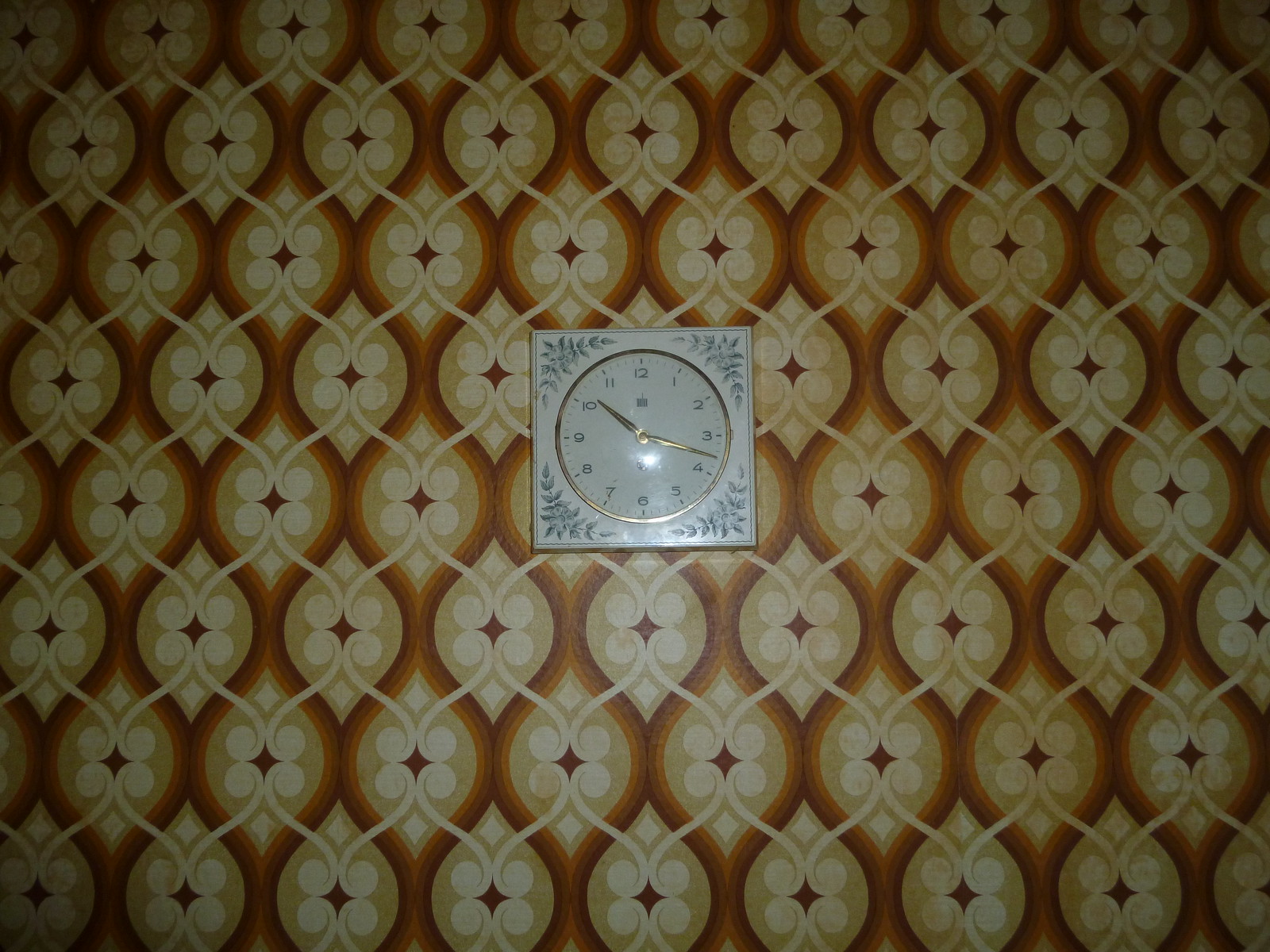The photograph features a wallpapered wall adorned with a central decorative clock. The wallpaper is a tan yellow with hues of white, browns, and oranges, forming a repeated geometric pattern of rounded diamonds framed by dark brown and intersecting curved lines in off-white. Each diamond hosts a four-petaled floral print with a dark brown center. At the top, the background melds into a lighter tan, enhancing the diamond shapes. Swirls are prominent on the sides and bottom, enveloping the entire wall in a complex, hourglass-like design.

Mounted slightly off-center, yet dominantly positioned in the middle, is a square clock. Predominantly white, the clock's face features a blend of gold and metallic silver accents. The hour and minute hands are metallic gold, complementing the dark gray to black Roman numeral-style numbers that mark the time as 10:18. The clock is bordered by light blue floral decorations and foliage patterns, likely resembling ferns, which embellish the corners and provide an elegant contrast to the geometric wallpaper. A gentle reflection shimmers on the clock face, adding a touch of realism to the scene.